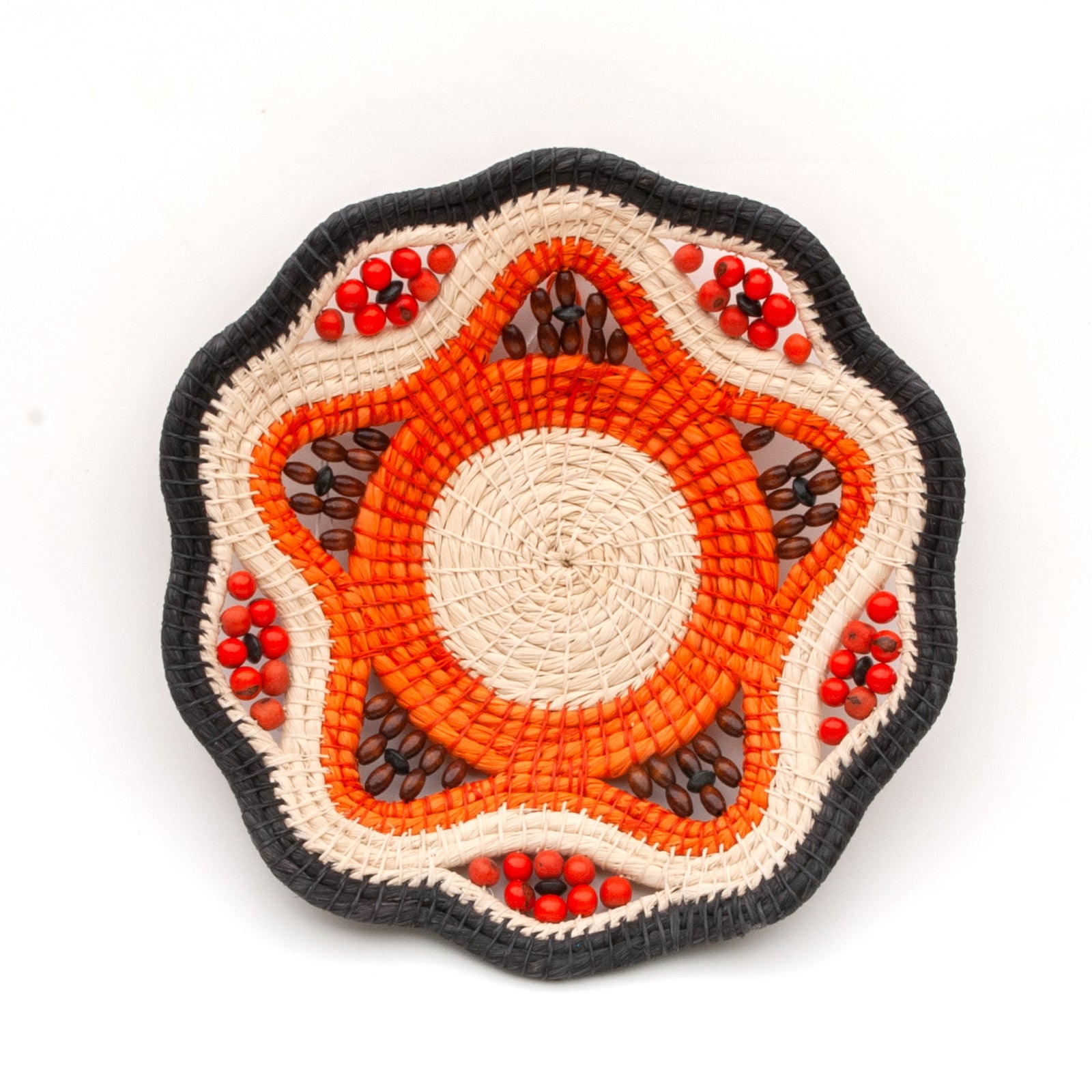This photograph, possibly taken indoors and with a stock photo aesthetic, features a handmade decorative item resembling a knitted or sewn fiber mat placed against a white background. The item showcases a unique circular design with an intricate wave-like black border that flows in and out. The main pattern alternates among light tan, red, and black colors, creating an eye-catching aesthetic. A central orange star is prominently featured, interspersed with round red beads on the outer sections and elongated brown oval beads in the inner sections, adding depth and texture. The star's core contains nested circles of orange and white, enhancing the ornate composition. The meticulous hand-stitching and varied thread colors harmoniously blend to create this artisanal piece, making it a compelling addition to home décor.